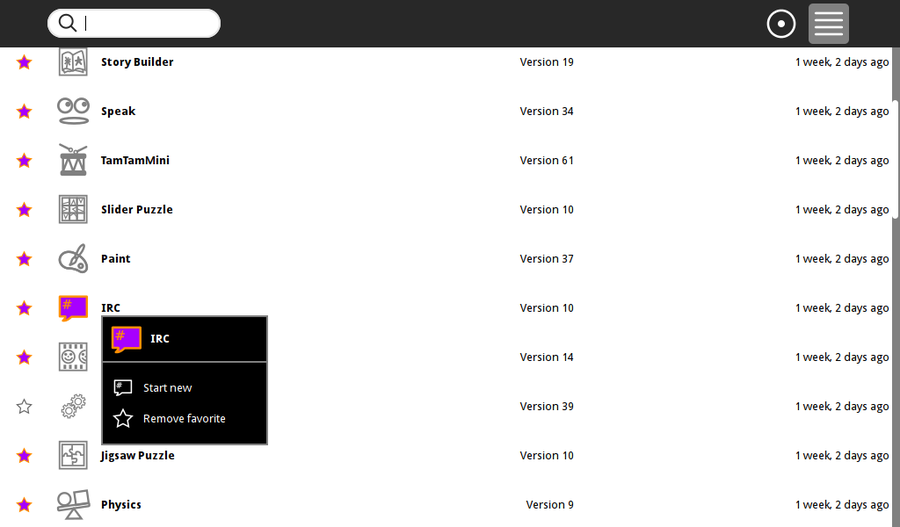The screenshot depicts various versions of an application system interface. At the top left corner, there is an empty search bar with a blinking cursor on the left side, indicating it is ready for user input. Directly beneath the search bar, the following options are listed: "Story Builder," "Speak," "TamTam Mini," "Slider Puzzle," "Paint," "IRC," followed by additional partially visible items obstructed by a pop-up box. 

The pop-up box, partially covering the options, displays text related to IRC, providing options to either "Start New" or "Remove Favorite." Below the pop-up with the partially visible options, the labels "Jigsaw Puzzle" and "Physics" are discernible. The layout suggests a structured directory or menu interface designed for varied functionalities, ranging from educational tools to utilities.